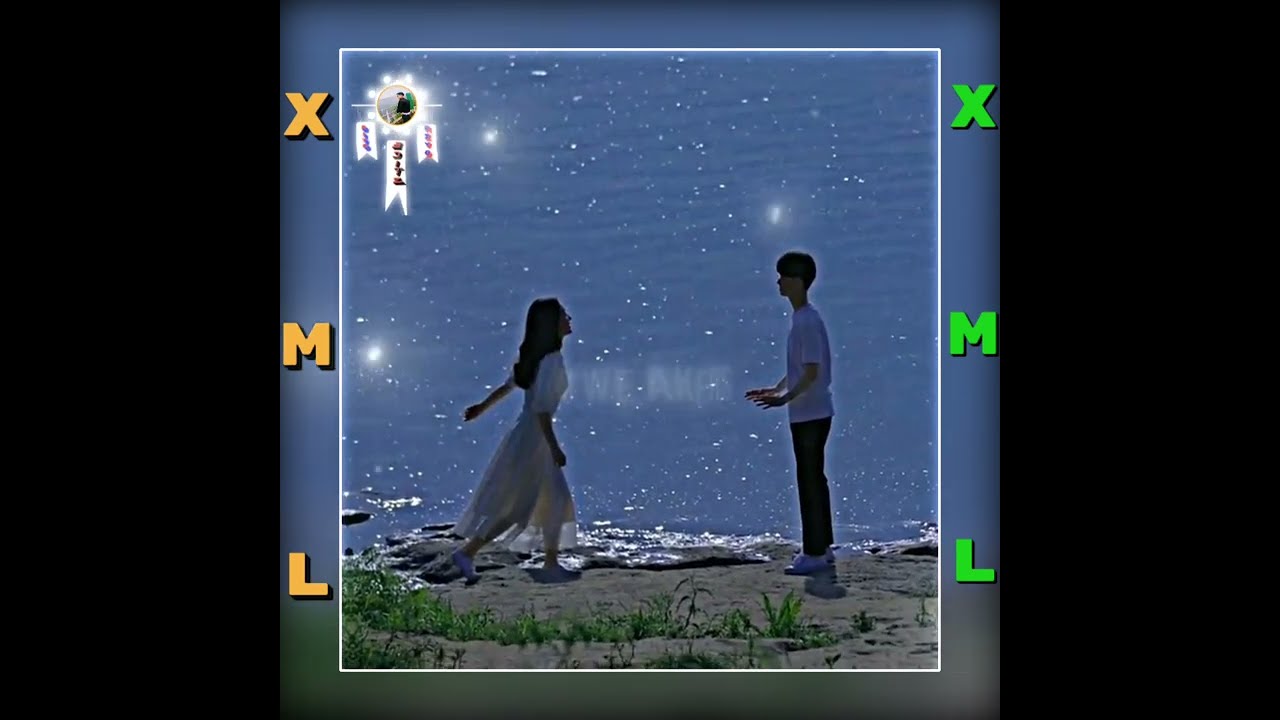The image appears to be an animated cover, likely for a music album. It features a romantic scene against a blue background. Dominating the cover are two young individuals, a man in a white t-shirt, black jeans, and white shoes, and a woman in a white dress, both with dark hair, standing on a dirt and rock formation interspersed with grass. They are gazing at each other under a starry night sky, near what seems to be an ocean with sparkling waves. The letters "XML" are vertically spaced on both sides of the image, with XML in yellow on the left and in green on the right. There is also a rectangular white square at the bottom framing the pair, adding a storybook-like effect. At the top left corner, a white ribbon logo is visible, contributing to the graphic's whimsical and romantic vibe.